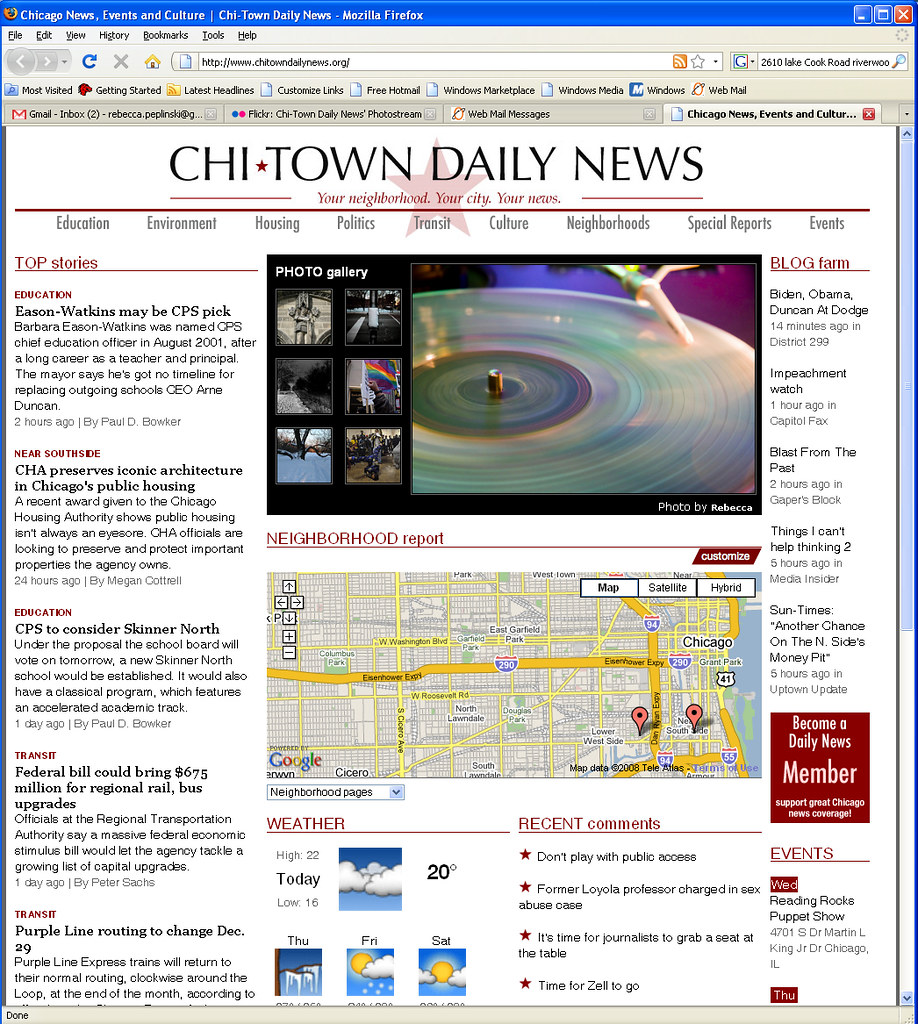Displayed in a Firefox browser window, this image showcases a website titled "Chicago News, Events and Culture" under the banner "Chi-Town Daily News," as indicated in the browser's title bar. In the upper right corner of the window, there are Minimize, Maximize, and Close buttons. The menu bar beneath features options such as File, Edit, View, History, Bookmarks, Tools, and Help.

The navigation bar includes icons for Refresh, Stop, and Home, followed by the URL www.chitowndailynews.org. Additionally, an RSS Feed button and a Google search bar are located on the far right. Below these elements, there are categorized bookmarks labeled Most Visited, Get Started, Latest Headlines, Customized Links, Free Hotmail, Windows Marketplace, Windows Media, Windows, and Webmail. Four browser tabs are open, showing Gmail, Flickr, Webmail Messages, and the Chicago News, Events and Culture website.

The main content of the webpage is set against a white background and comprises diverse headlines and articles from the Chi-Town Daily News, emphasizing their slogan: "Your Neighborhood, Your City, Your News." Categories such as Education, Environment, Housing, Politics, Transit, Culture, Neighborhoods, and Special Reports and Events are prominently displayed. A photo gallery is featured, with one image displaying a vinyl record playing on a turntable. Additionally, there is a map highlighting a local neighborhood, complemented by today's weather details: 20 degrees Fahrenheit with a high of 22 and a low of 16 degrees.

On the left-hand sidebar, several top stories are listed, including:

1. Education: Eason Watkins May Be CPS Pick, Near South Side
2. SCH Preserves Iconic Architecture in Chicago's Public Housing
3. Education: CPS to Consider Skinner North
4. Transit: Federal Bill Could Bring $675 Million for Regional Rail and Bus Upgrades
5. Transit: Purple Line Routing to Change December 29th

The right-hand sidebar features categories such as Blog Forum, with posts titled:

1. Biden, Obama, Duncan at Dodge
2. Impeachment Watch
3. Blast from the Past
4. Things I Can’t Help Thinking
5. Sometimes Another Chance on the Inside's Money Pet